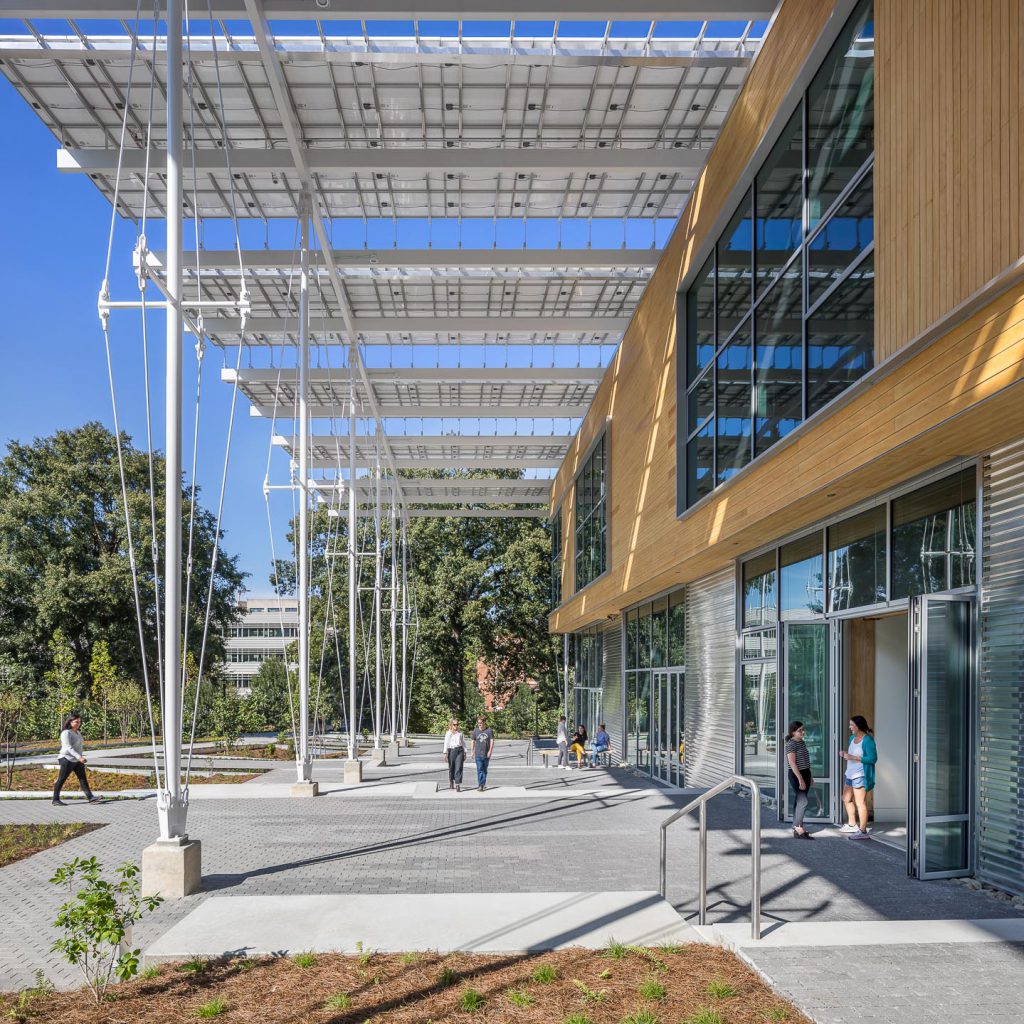The image features a large, modern building composed of wood, metal, and ample windows. The upper right side exhibits narrow vertical slats of wood, accompanied by a prominent rectangular window centrally located. Below, there is a section of horizontal wood slats forming a hipped roof. The lower right corner showcases large glass doors, with two women conversing in the doorway—one in a green jacket, the other in a striped t-shirt. The entrance is subtly elevated by a couple of stairs, featuring a short metal railing at the center.

A mixture of gray bricks and brown grass with green weeds make up the ground, along with a green bush in the lower left. Several individuals populate the scene: two people walk towards the observer from the background, a group sits and stands at a table to the right, and a lady approaches the entrance from the left. The walkway before the building is shaded by protruding roof panels, supported by poles embedded in concrete blocks, which allow glimpses of the clear blue sky above. In the background, large trees further accentuate the idyllic setting.